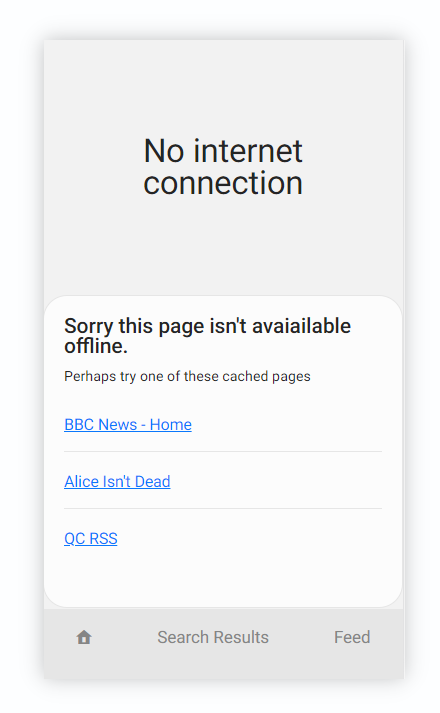The image displays a web browser page with an error message indicating that there is no internet connection. The message reads, "Sorry, this page isn't available offline. Perhaps try one of these cached pages." Below the message, there are three hyperlinks rendered in blue: "BBC News Home," "Alice Isn't Dead," and "QC RSS." At the very bottom of the page, there are small icons or buttons labeled "Home," "Search Results," and "Feed," suggesting navigation options within offline content or cached items.